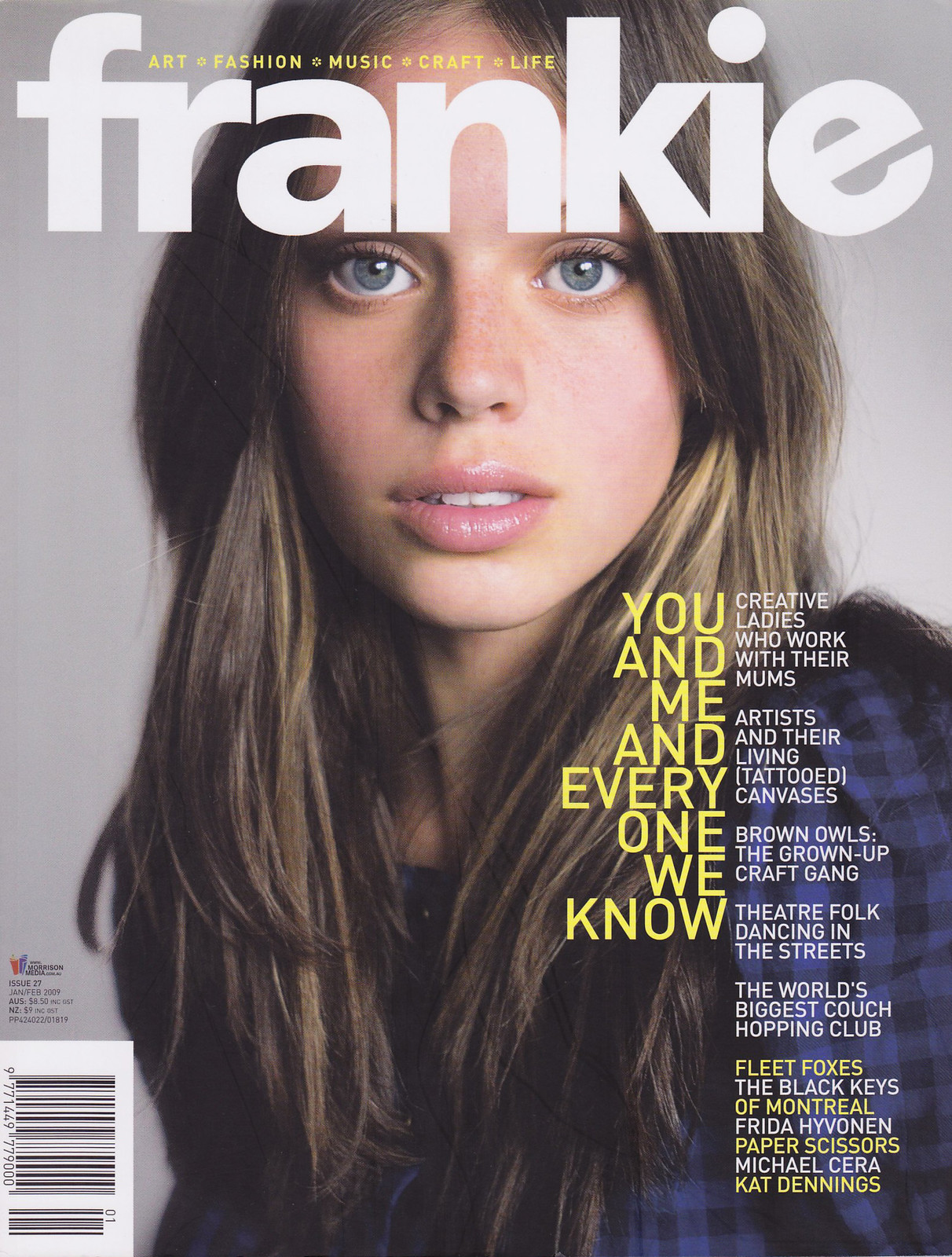The magazine cover features a young woman with long, chest-length dark brown hair accented by blonde highlights, big blue eyes, and pink lips. She wears a blue and black striped flannel shirt, revealing some of her shoulders and chest. Her expression is innocent, with her mouth slightly open and freckles visible on her nose, as she gazes directly into the camera. 

At the top of the cover, in small yellow all-caps, it reads “ART, FASHION, MUSIC, CRAFT, LIFE.” Below this, the title "Frankie" is boldly displayed in large white lowercase letters. On the lower right side, a prominent caption in white reads “You, Me and Everyone We Know,” followed by article highlights in varying colors including yellow and white. These articles cover topics such as creative ladies working with their mums, artists and living tattooed canvases, and brown owls to craft gang theater folk dances. Other highlights include features on bands and artists like Fleet Foxes, The Black Keys, Of Montreal, Frida Hyvönen, Paper Scissors, Michael Cera, and Kat Dennings.

In the bottom left corner, there is a barcode with additional details: “Issue 27, Jan-Feb 2009, Morrison Media, Aussie $8.50 including GST, New Zealand $9 including GST, PP 424022/01819.” The background of the cover is a light blue or gray color.